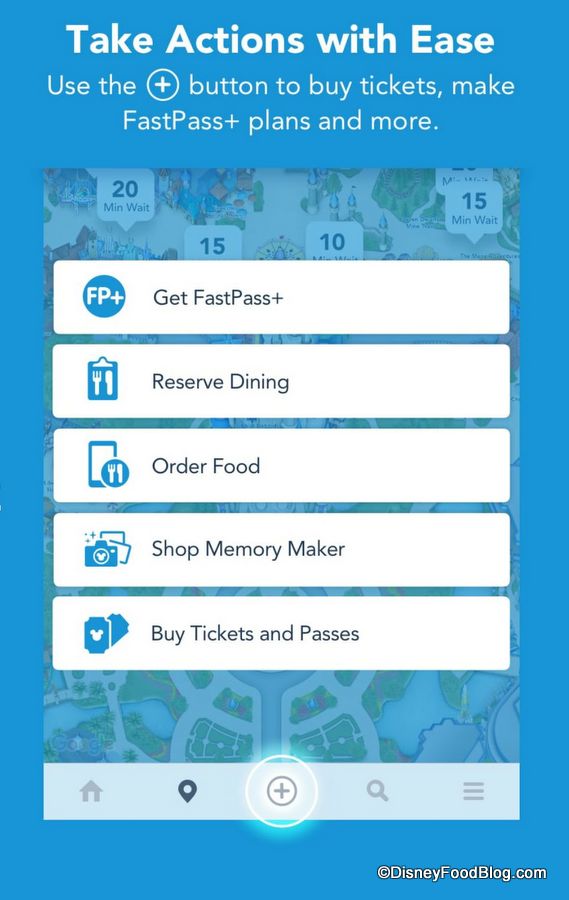This image is a screenshot from DisneyFoodBlog.com, showcasing a section of the Disney app. The interface has a blue background with a prominent banner at the top that reads, "Take actions with ease. Use the plus button to buy tickets, make FastPass+ plans, and more." Below this banner, a faint image of one of the Disney parks serves as a subtle backdrop, possibly depicting the Magic Kingdom, though it is not clearly identifiable.

Stacked vertically in the center, there are five interactive white buttons, each offering a different feature for users:
1. Get FastPass+
2. Reserve Dining
3. Order Food
4. Shop Memory Maker
5. Buy Tickets and Passes

At the bottom of the screen, just above the DisneyFoodBlog.com watermark in the bottom right corner, are five icons: a home icon, a locate icon, a plus icon, a search icon, and a menu icon with three dots, providing quick access to various functionalities of the app.